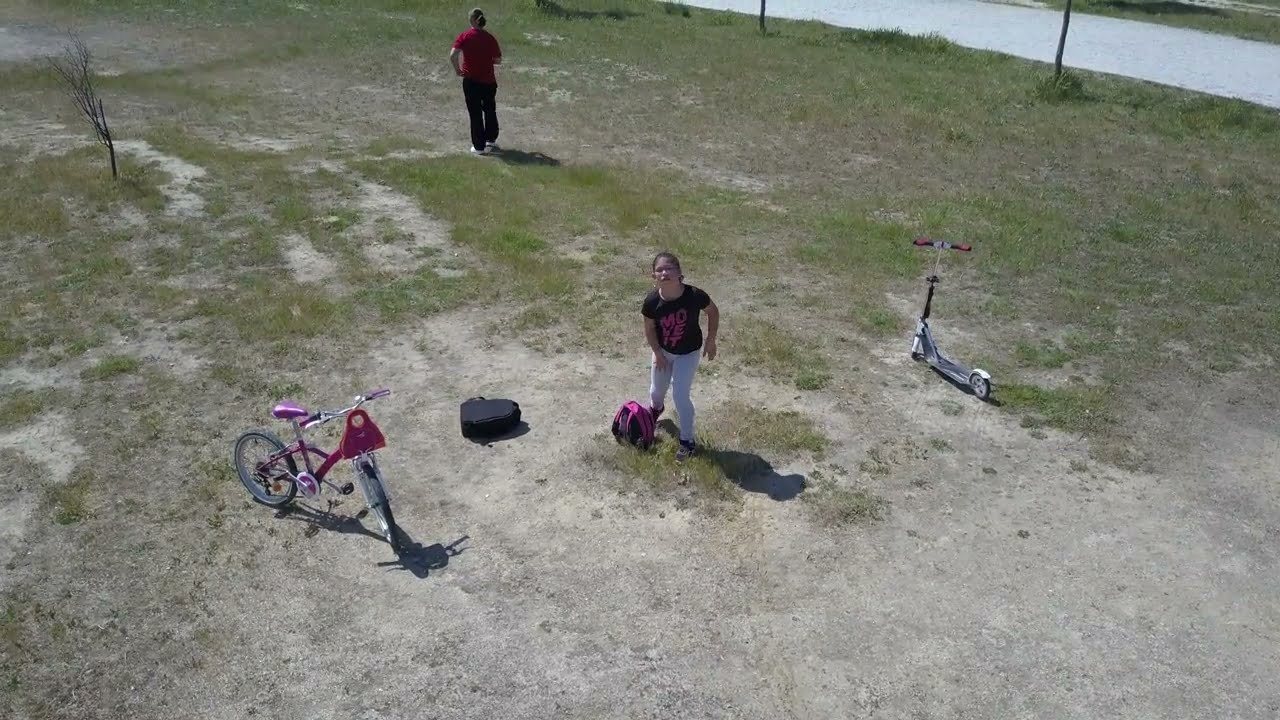The image features a dry, grassy area blending into patches of dirt, set in an arid environment. At the lower left, there's a children's pink and white bike. Towards the center right, a basic hand-riding scooter is visible. Central to the image, a girl stands holding a green towel, her pink bag resting on the ground nearby. She appears to be looking down. Just behind her, an adult male dressed in a red shirt and black pants is absorbed in his phone. The scene includes various colors, such as pink, gray, black, white, light blue, red, tan, and purple, indicating the mid-day sunlight. The backdrop hints at an outdoor setting, possibly a park, with the ground primarily dirt near the bottom and transitioning to grassy towards the top.